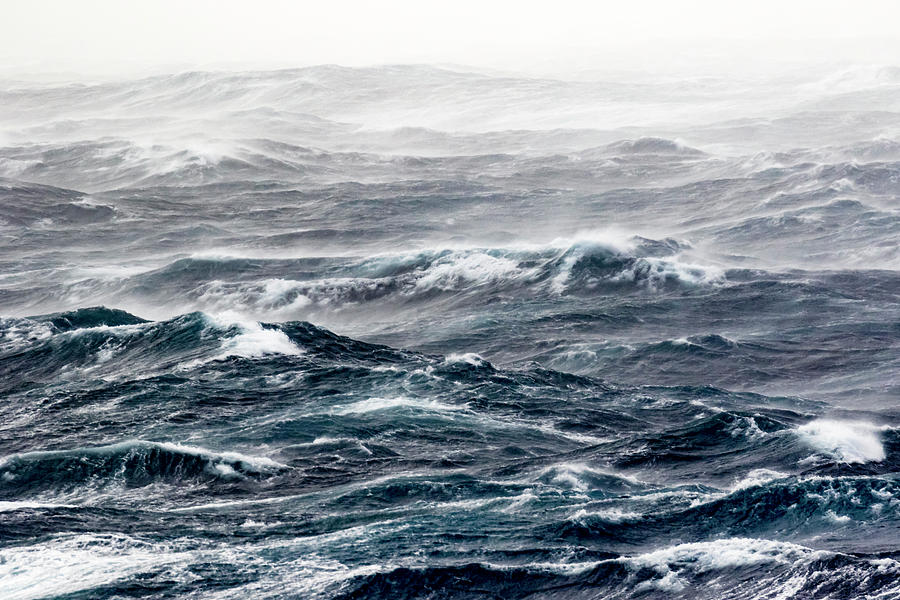The image captures a tumultuous ocean scene with choppy, rocking waves. In the foreground, the water is a crystalline blue, transforming into a dark, bluish-black hue as it extends to the background. The waves are turbulent, with numerous white caps crashing and creating a fine sea spray that produces a white mist above the water. The atmosphere is stormy and cold, accentuated by a greyish, foggy sky that hints at incoming severe weather. The scene is devoid of any boats, fish, or humans, emphasizing the raw, natural power of the stormy sea.